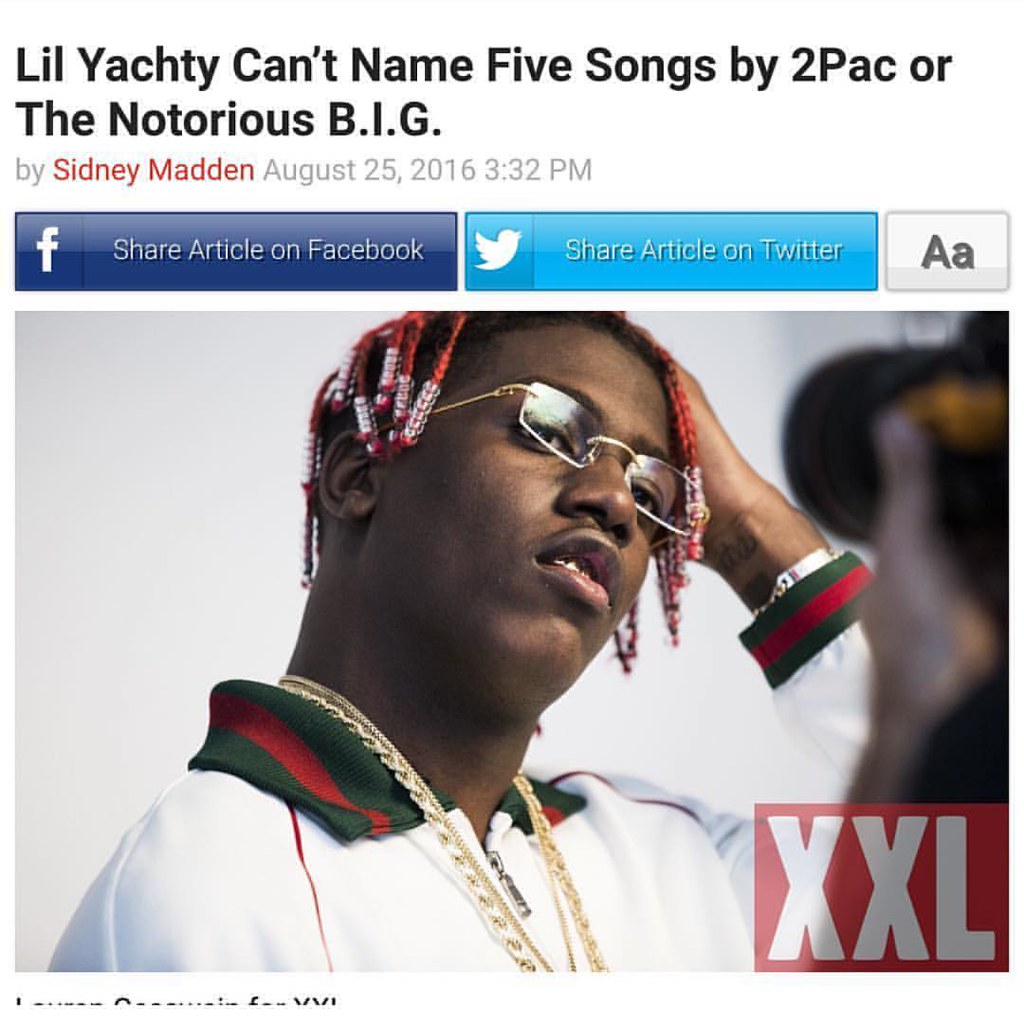In this Instagram post, dated August 25, 2016, at 3:32 PM and written by Sidney Madden, a headline reads, "Lil Yachty Can't Name Five Songs by Tupac or the Notorious B.I.G." The image features rapper Lil Yachty with his distinctive red cornrows adorned with beads, styled into braids. He wears a white Gucci zip-up shirt, marked by the iconic red and green Gucci logo on the collar and sleeve ends, complemented by an ID bracelet and multiple gold chains that hang around his neck. Adding to his distinctive style, Lil Yachty sports glasses and appears to have a somewhat confused expression, with his hand resting on his head. In the corner of the image, the logo “XXL” is visible. In addition, below the headline, the text includes sharing options with Facebook and Twitter logos, as well as lowercase and uppercase text size options for the article.